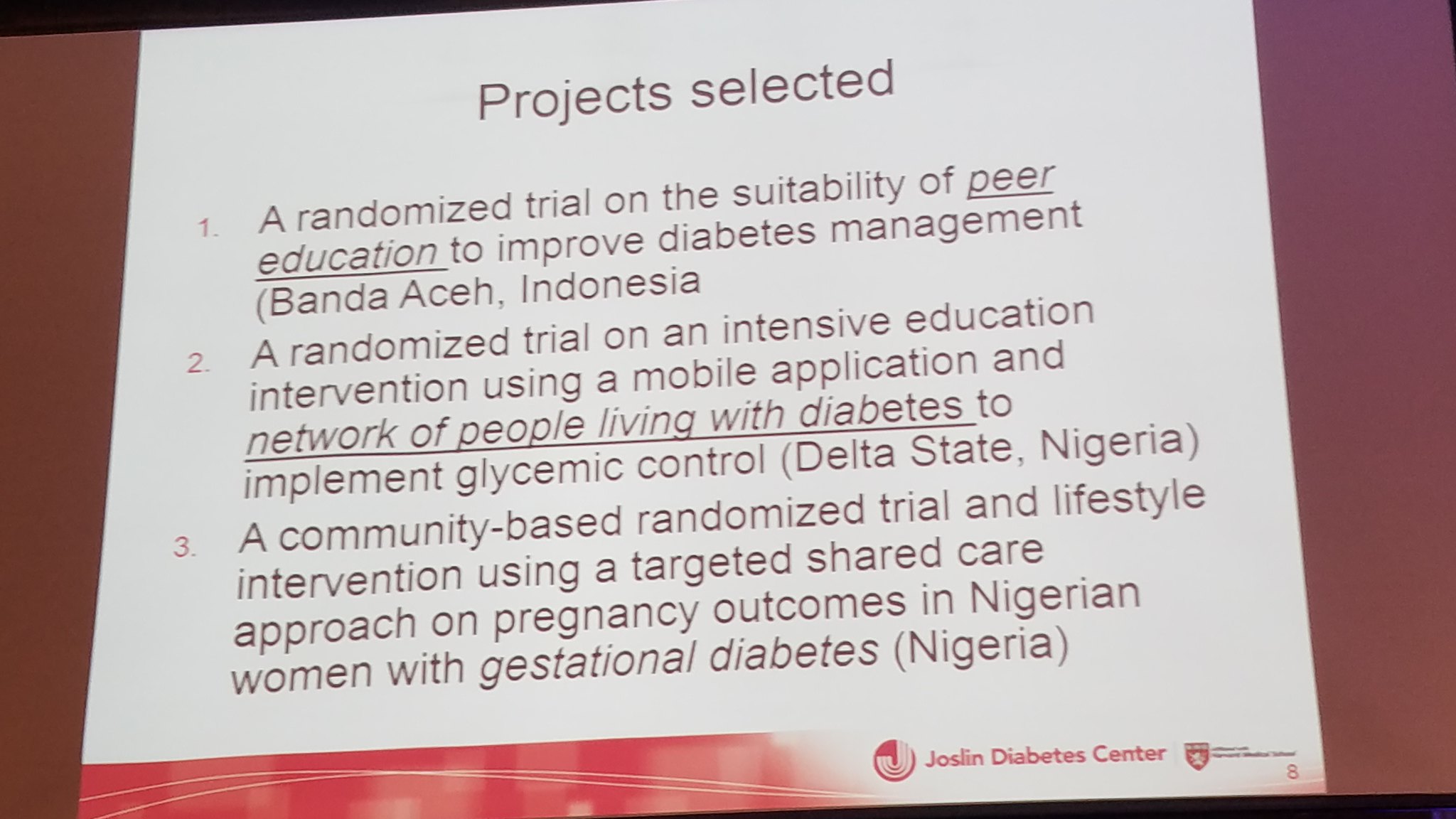The image depicts a close-up of a projected presentation slide with a white background and dark text. The slide, rectangular in shape, features a heading that reads "Project Selected," indicating the discussed topic is about diabetes management. The slide contains three main points enumerated by reddish numbers on the left side. Here are the points in detail:

1. A randomized trial on the suitability of peer education to improve diabetes management.
2. A randomized trial on an intensive education intervention using a mobile application and a network of people living with diabetes to implement glycemic control.
3. A community-based randomized trial and lifestyle intervention using a targeted shared care approach on pregnancy outcomes in Nigerian women with gestational diabetes.

The text of these points is smaller than the heading. At the bottom of the slide, there is a red graphic footer along with the logo of the Jocelyn Diabetes Center. The slide borders are darker, likely indicating the screen boundaries surrounding the projected image.